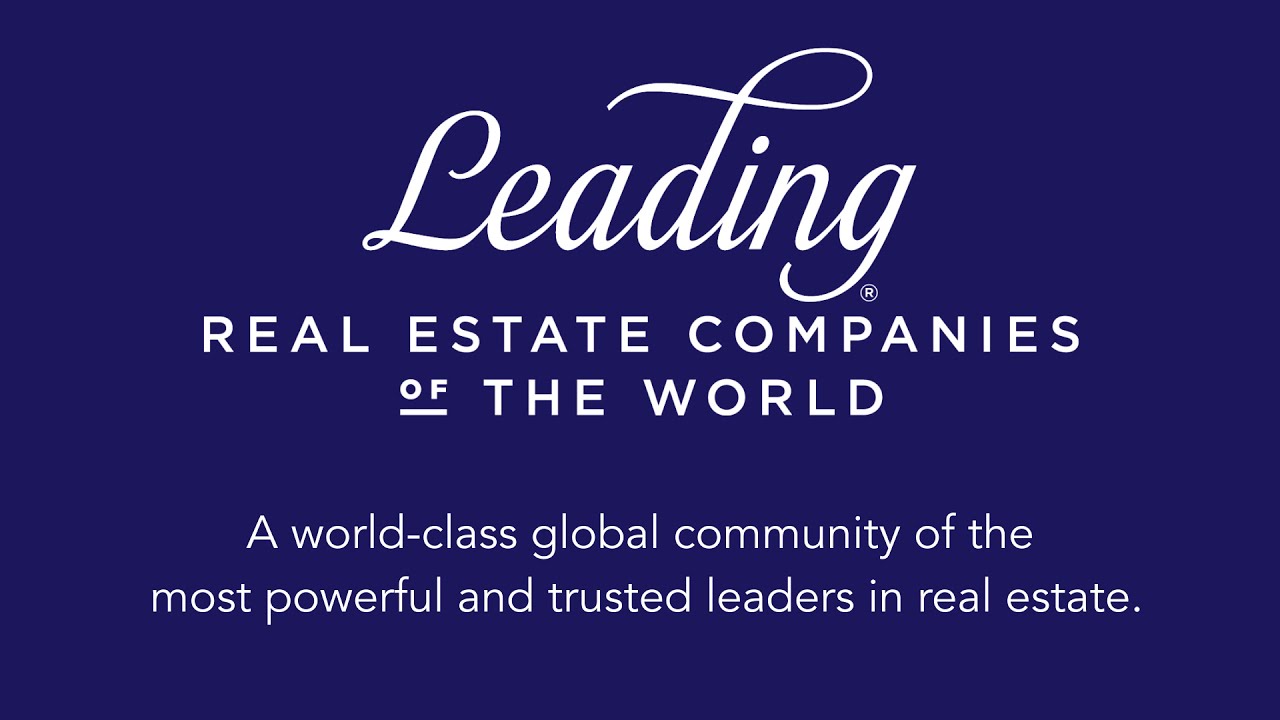This horizontal, rectangular image features a solid, brighter dark blue background. The centered text across the image is all in white, with varying font sizes. At the top, the word "LEADING" is written in cursive, with a trademark symbol (®) nestled under the 'G'. Below, in slightly smaller all-caps white font, the text reads "REAL ESTATE COMPANIES OF THE WORLD," with the word "OF" being smaller and underlined. At the bottom of the image, in even smaller white print, it says, "A WORLD-CLASS GLOBAL COMMUNITY OF THE MOST POWERFUL AND TRUSTED LEADERS IN REAL ESTATE." The text is neatly centered and there are no images or icons present. The overall impression is that this might be an informational card or an advertisement for a well-regarded real estate organization.